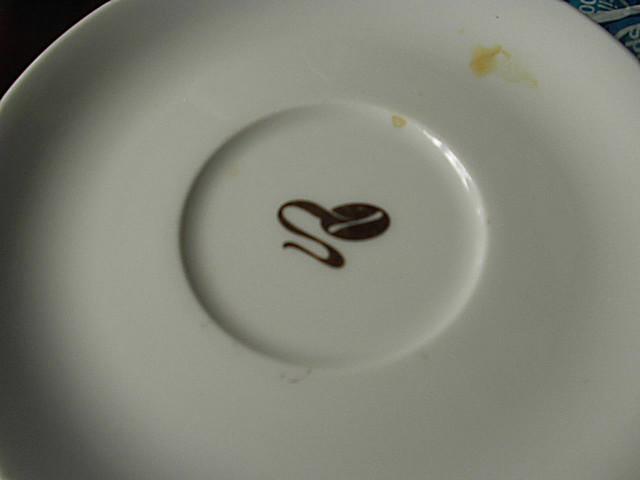The close-up image depicts a white porcelain item, likely the underside of a plate or a saucer, characterized by its circular shape with visible arcs in two corners of the frame. At the center of this circular object is a raised, dome-like logo that resembles a stylized coffee bean with a wisp of aroma, depicted in dark brown or black. This central logo also has an S-shape with a circular element that includes a white line through it. The plate or saucer has evident signs of wear, with small yellowish-brown stains, possibly rust or coffee, concentrated in the upper right area. There is also a faint blueish pattern, which might be from an underlying fabric visible in the top right corner. The background suggests the item is resting on a tablecloth. Overall, the image emphasizes the unique central logo and the dish's slightly dirty condition, hinting at its use in a coffee or tea setting.